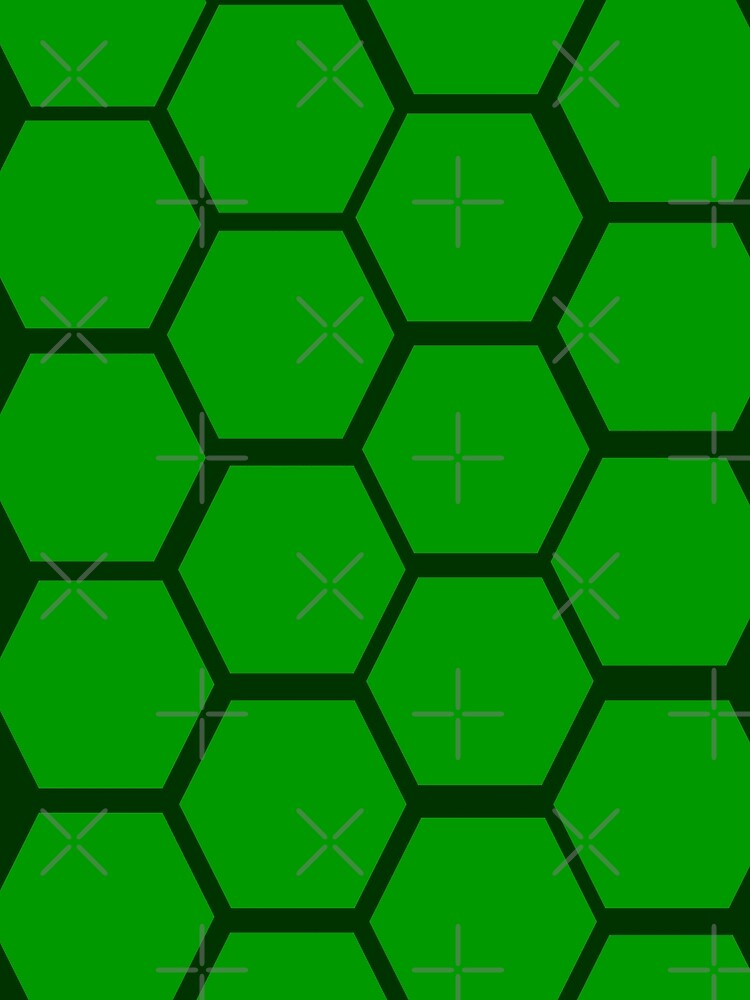The image features a distinctive honeycomb pattern composed of bright lime green hexagons arranged in a grid formation. There are four visible columns, each containing five hexagons. The hexagons are outlined by narrow, very dark green lines, which are almost black in appearance. This dark green forms the background and the framework for the pattern. Overlaying the hexagonal design is a translucent watermark consisting of repetitive plus signs and X symbols, each missing their centers. These symbols appear in a light gray color and are systematically distributed across the image, creating an intricate secondary pattern that overlays the vibrant lime green hexagons and the dark green background. The overall effect is a complex and visually engaging geometric design.